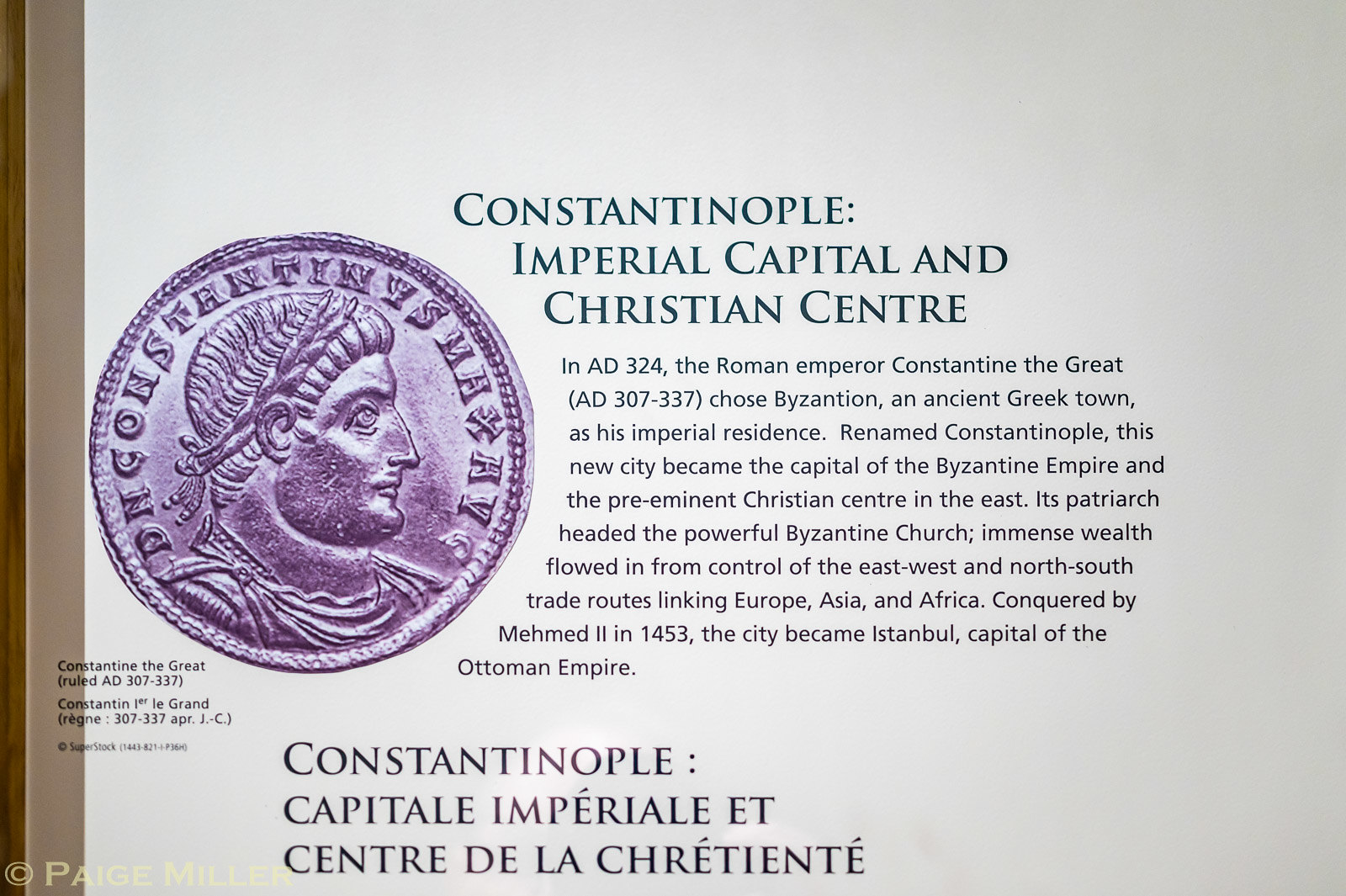The image is a professionally designed slide from a PowerPoint presentation with a clean, white background. On the left side of the slide, two vertical brown lines run from the top to the bottom, with the thinner line on the very edge and the thicker line slightly inward. In the bottom left corner, the yellow font reads "© Paige Miller."

Prominently displayed on the left side is a large, purplish silver coin featuring ancient language and the side profile of a person wearing a wreath crown, identified as Constantine the Great, who ruled from AD 307 to 337. 

To the right of the coin, the title "Constantinople: Imperial Capital and Christian Center," is shown in all caps, spanning three lines. Below the title, the body text discusses how Roman Emperor Constantine the Great, in AD 324, selected the ancient Greek town of Byzantium as his imperial residence and renamed it Constantinople. This city subsequently became the capital of the Byzantine Empire. The text curves slightly to match the curvature of the coin.

The section is likely a print or promotional piece that could be used in a museum exhibit or historical presentation, showcasing sophisticated graphic design elements.